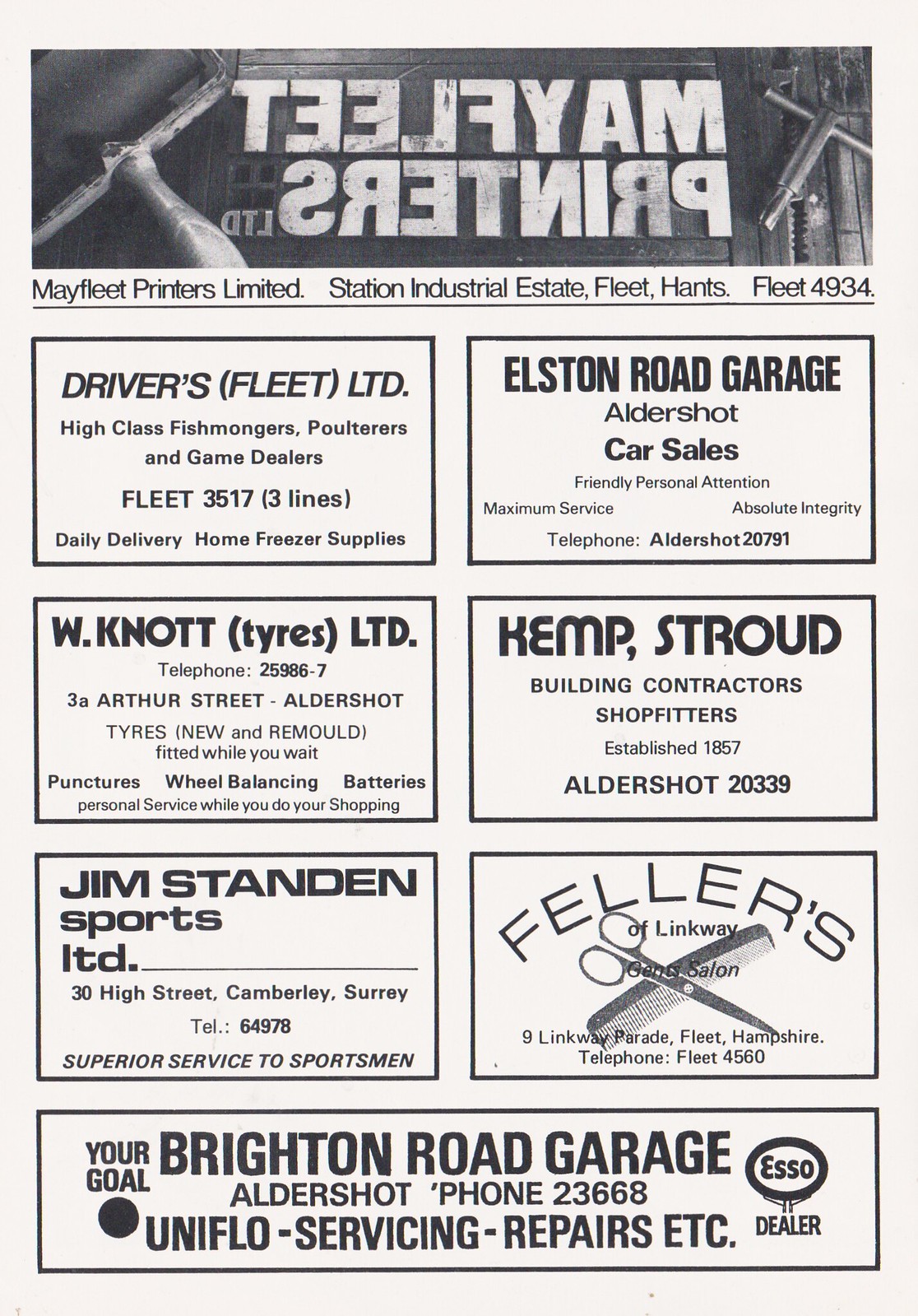The image is a black-and-white advertisement page featuring multiple ads, primarily for local businesses. At the top, there's a notable mirrored text reading "Mayfleet Printers Ltd" with the address "Station Industrial Estate, Fleet, Hants, Fleet 4934" in white font. This section also includes an image, possibly depicting tools like a paint roller. Beneath this header, there are seven rectangular ads arranged in three rows of two and one larger rectangular ad at the bottom. The businesses advertised include:

1. **Drivers Fleet Ltd**
2. **Elston Road Garage**
3. **W. Nought Tyres Ltd**
4. **Kemp Stroud Building Contractors**
5. **Jim's Tandon Sports Ltd**
6. **Fellers of Linkway (possibly a salon)**
7. **Brighton Road Garage (an Esso dealer offering servicing and repairs)** 

Each ad contains detailed information about services, contact details, and other pertinent info specific to the businesses. The overall design features a white background with bold black text and bordered sections for each advertisement, giving the page a structured appearance.